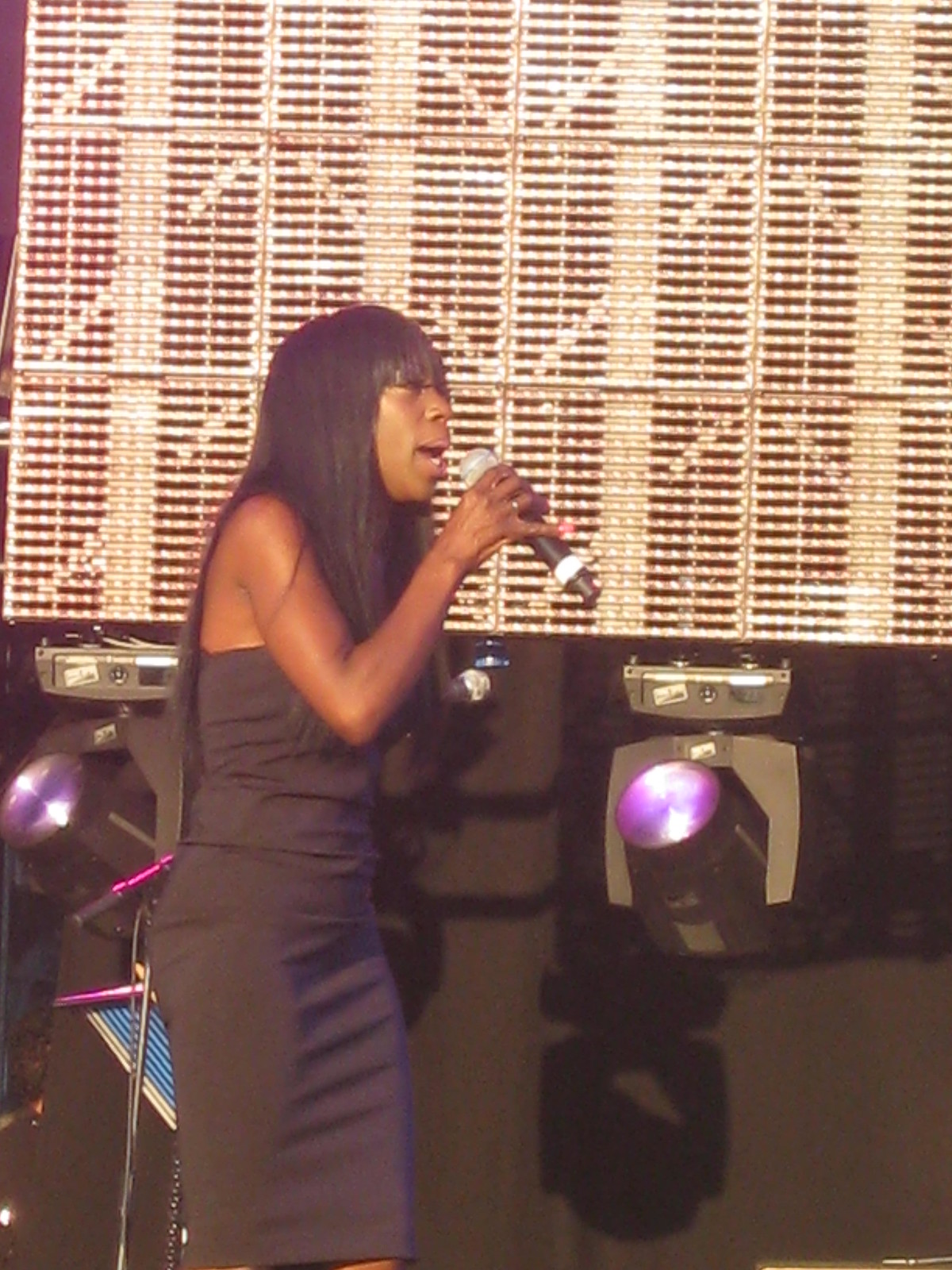The image captures a black woman with long, straight black hair and bangs that extend to her eyes, standing in profile on a stage. She is mid-performance, singing into a black microphone held in her right hand, with her pinky finger prominently extended, showcasing a pink-painted nail. She is attired in a form-fitting, strapless black dress, which reaches down past her knees, suggesting a stylish and elegant appearance. Her surroundings include various pieces of stage equipment and a backdrop featuring gold horizontal slats interspersed with black spaces, creating a slatted pattern. To her left and right, upwards-pointing purple stage lights cast a vibrant hue on the scene, while shadows and potential stereo or karaoke equipment are faintly visible against the black floor. The overall ambiance suggests an electrifying musical performance, possibly captured from the audience's perspective.